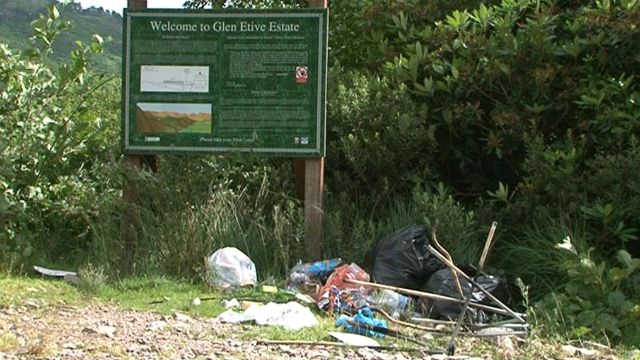The image depicts an outdoor scene dominated by a horizontally aligned rectangular sign attached to a wooden pole. The sign, situated towards the center-left of the photo, features a green background with a gray border and white text that reads "Welcome to Glen Etive Estate." The sign also displays two rectangular images: one resembling a map and the other a picture of a mountainous area, accompanied by extensive small text which is illegible due to the distance. The background is lush with dense trees, particularly thick on the right, and some distant trees visible in the upper left corner, suggesting they may be on hills or a mountain. The ground in the foreground is strewn with various types of garbage, including several large black bags, white bags, blue bags, a red bag, and numerous sticks jutting out of the dirt or rocky surface, indicating the area in front of the sign has unfortunately become a dumping ground.